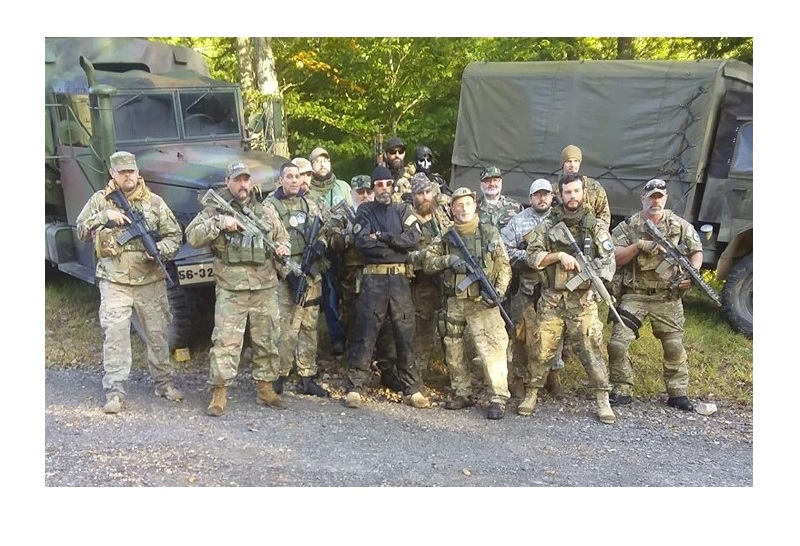In this photo, there is an army unit consisting of approximately 15 to 20 military men standing on a gravel road. The background features two green military trucks with their beds covered by large pieces of canvas, and beyond them, a wooded area with trees and grass. The men are mostly dressed in green camouflage uniforms and are carrying rifles pointed toward the ground. They are equipped with a variety of helmets and some wear vests with additional pockets. At the center of the group stands a man distinctively dressed in black slacks, a long-sleeve black shirt, and a black ski beanie-type cap, with a gray or green utility belt. This man also has sunglasses, a beard, and a mustache. Additionally, there are a few other figures in black towards the back, including one with a noticeably white face resembling a skeleton mask, and another with a long black beard and dark sunglasses. The composition of the scene captures the military unit in a calm, yet regimented posture against the backdrop of the vehicles and natural surroundings.